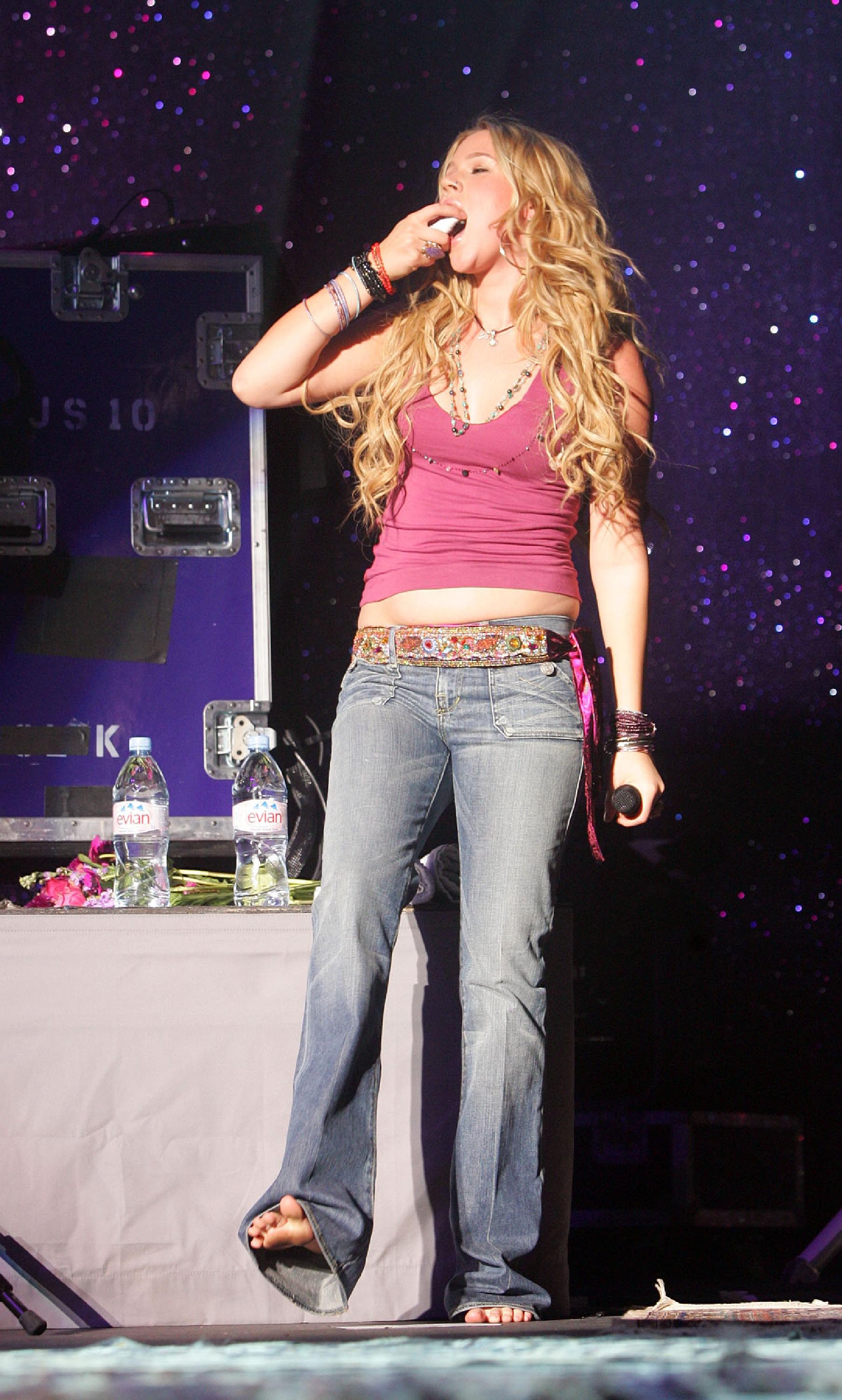In this image, a singer is captured mid-performance on stage. She holds a microphone in her left hand while her right hand is poised near her mouth, possibly using a breath spray. She is confidently raising her right leg straight into the air, with her left foot firmly on the ground. Her outfit consists of blue jeans with a floral belt and a pink tank top, and she is barefoot. The singer’s long, flowing blonde hair cascades down her shoulders, and her wrists are adorned with numerous wristbands and bracelets. The stage behind her is decorated with a sparkling, purple, glittery backdrop, creating a star-like effect. To her right, there is a table with two water bottles and some pink flowers, as well as a compartment with silver lock mechanisms. A sign in the background, possibly reading "US 10," adds to the ambiance of the performance setup.